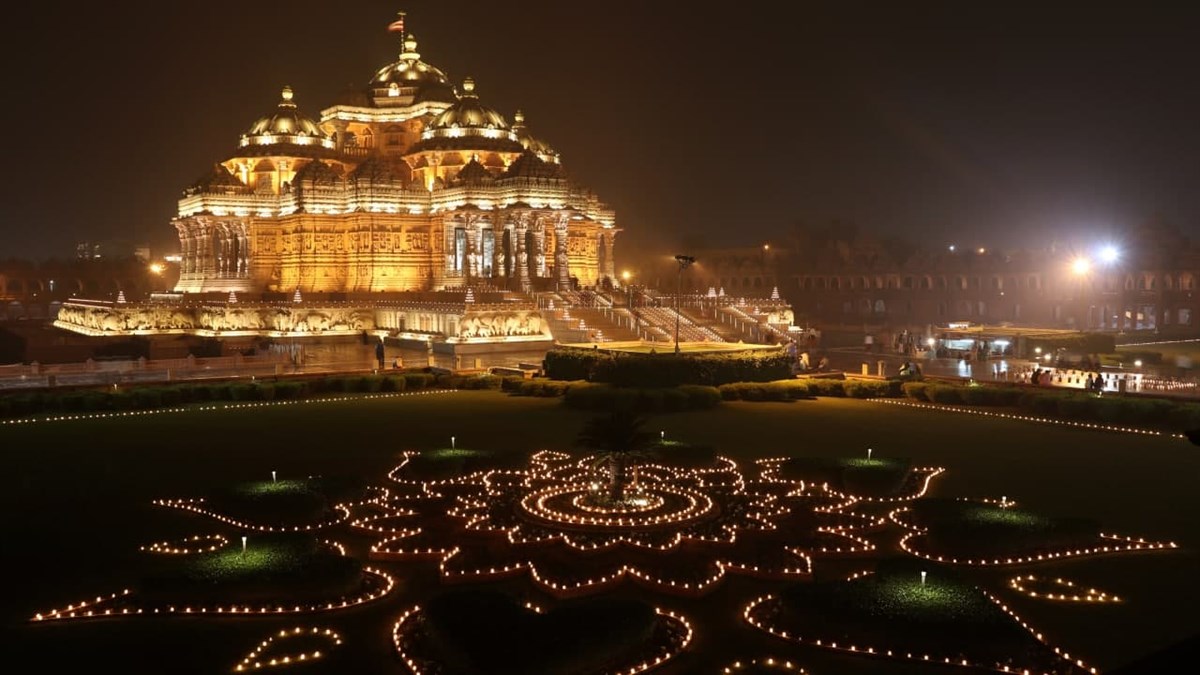This nighttime photograph showcases a large, ornate building, possibly a temple or palace, illuminated with an intricate array of lights. Dominated by intricate architecture, including at least three domed roofs and several columns at the grand entrance, this majestic structure is highlighted in creams, oranges, and light browns. The American flag prominently flies from its highest dome, reinforcing its potential location in the United States. In the foreground, a carefully manicured lawn features green shrubs and a striking light design resembling a lotus flower with petals and leaves, enhancing the nighttime beauty. Surrounding this central building is a lower, brownish structure on the right, almost overshadowed by the grandeur of the main edifice. The grand staircase leading from the building's entrance descends to a vast plaza, adorned with hedges and a concrete courtyard. Rows of less illuminated buildings can be seen in the background, adding depth to the scene.